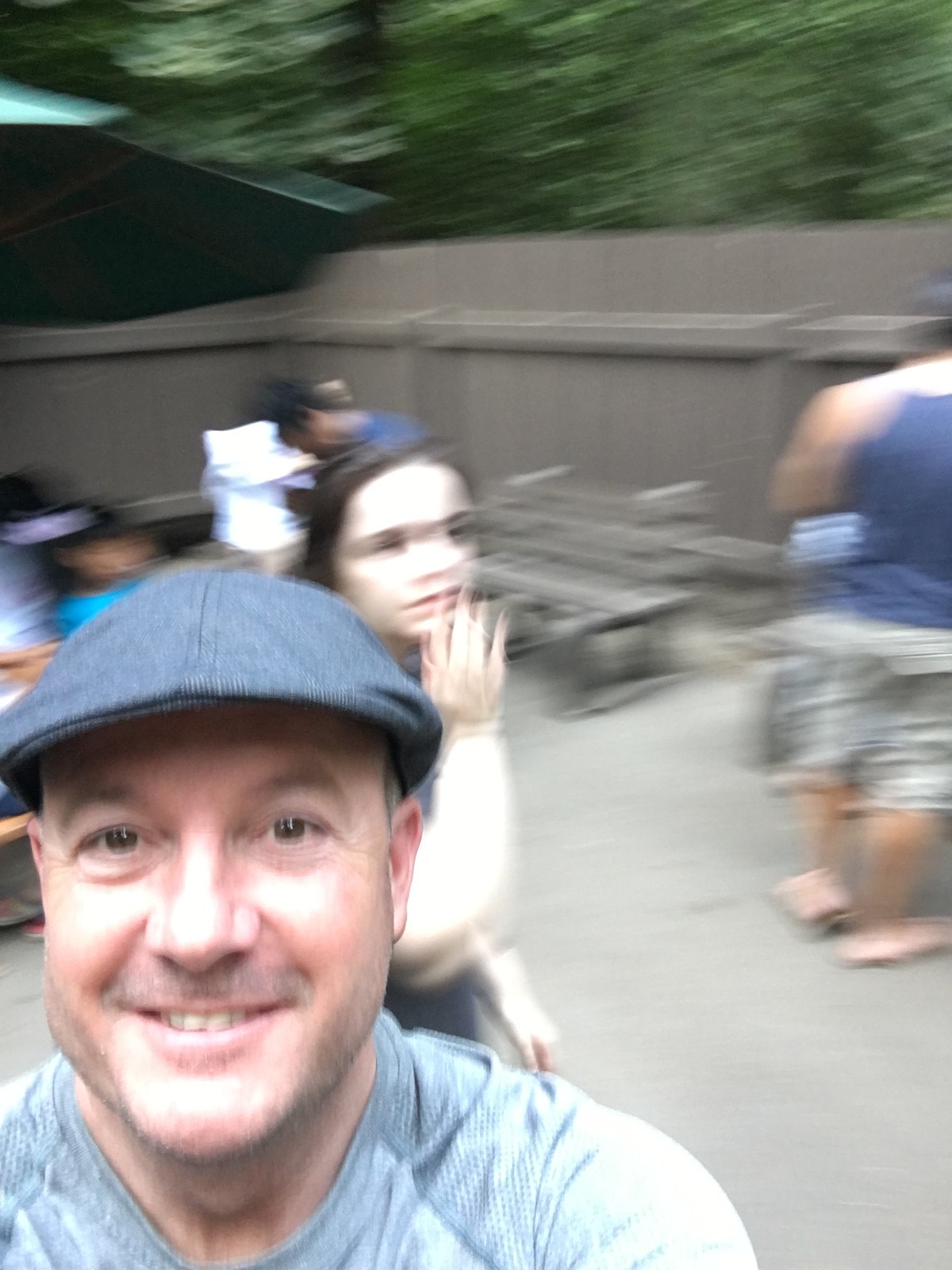In this vertically-oriented photograph, most of the image is blurred, except for the lower left corner. Here, a man in his early 40s is clearly visible from the shoulders up, wearing what appears to be a light blue or light gray crew neck shirt. He is smiling warmly with brown eyes and has a slight five o'clock shadow on his beard and mustache. The man is also wearing a blue cap. 

Behind him is an extremely blurry figure of a woman with brown hair, visible from the waist up, who appears to have her hand up to her mouth. Both individuals are Caucasian. In the lower and upper right corners of the image, there is the back of a male figure in shorts and a tank top, standing against a fence. The background features a sunlit scene with a few picnic benches and what seems to be a human head barely visible. The photograph is clearly taken during the daytime under bright lighting conditions.